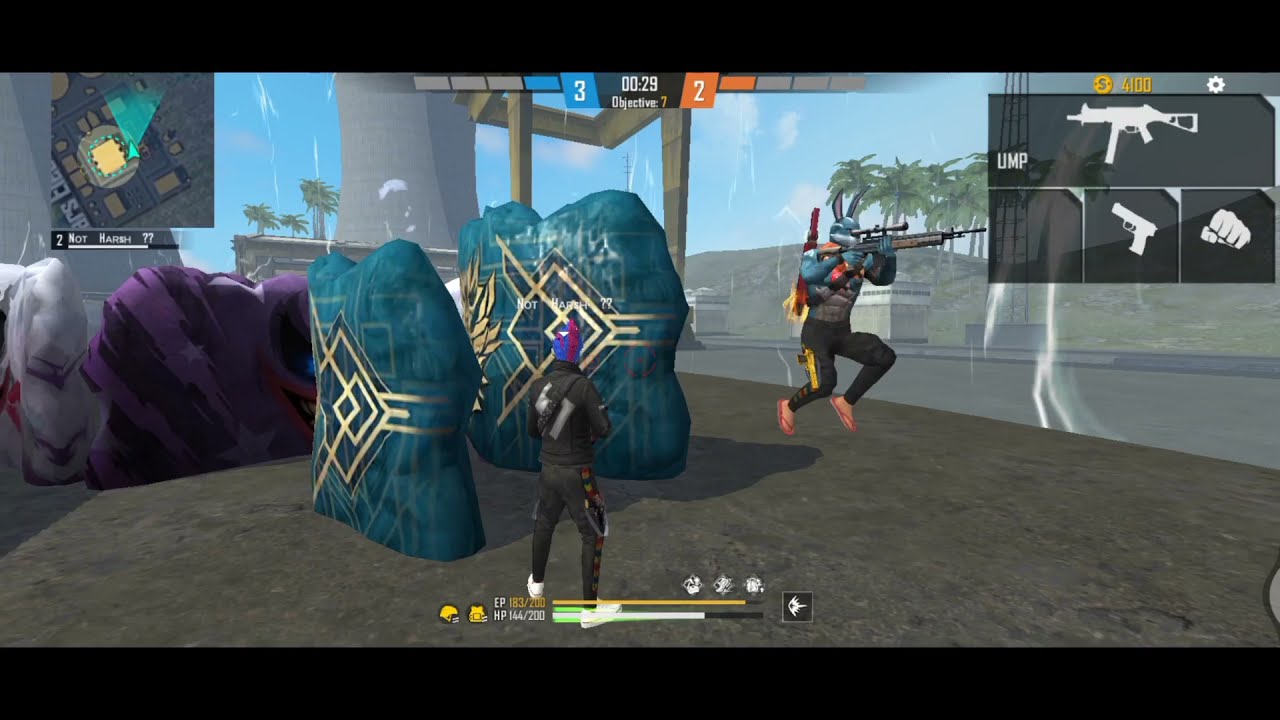This image is a detailed screenshot from a video game featuring a vibrant scene with various elements. The screen is bordered by black bars at the top and bottom, and there’s a black box to the right displaying a picture of a rifle, a handgun, and a fist labeled "UMP" with a gold dollar sign above it reading "$400." Central to the image, the top shows a score of "3" in blue and "2" in orange, alongside a timer set at "00:29." Two action characters dominate the scene: one stands facing away in the middle, darkly dressed with white shoes and possibly equipped with a helmet and something held over his shoulder. The other character, also darkly dressed, is airborne, wearing reddish shoes, and appears to be firing a rifle while another weapon is visible on his back. Below these characters, there are yellow and white bars accompanied by various icons.

On the left, large, colorful stones can be seen—two blue, one purple, and one white—standing distinctively against the backdrop. The background extends into distant small hills, tall concrete and wooden structures, and lush palm trees under a clear blue sky. An upper-left diagram, potentially a map, includes some small text beneath it, while the upper-right corner contains options for different weapons with another small icon and yellow writing above it. This richly detailed scene intricately blends in-game elements with detailed environmental features, illustrating a dynamic moment of gameplay.